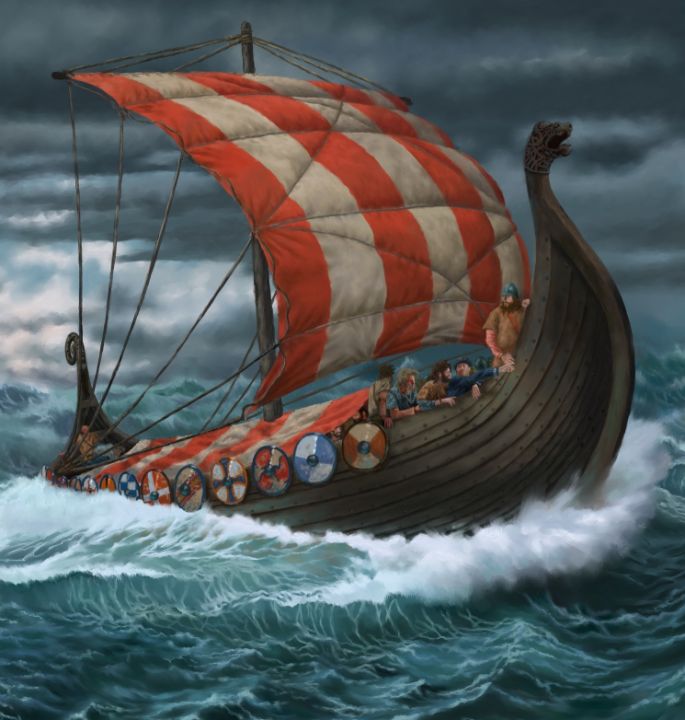This detailed illustration portrays a Viking ship navigating through tumultuous, greenish-blue seas, with large waves crashing against the vessel, creating white froth around it. The ship is seen in profile, moving from left to right, with the bow prominently adorned with an intricately designed dragon's head. At the stern, the tail of the same dragon design is seen, complementing the ornate craftsmanship.

The ship has a single large sail that is patterned with alternating red and white stripes, held in place by multiple ropes extending from the back of the ship. A striped canopy, matching the sail's design, covers part of the interior. Numerous round shields line the right side of the boat, displaying various designs in blue, tan, and white.

Onboard, six Viking men are depicted. One is positioned at the head, broad and attentive, wearing a Viking hat, while others are engaged in conversation or gazing out to sea. The stormy sky above mirrors the rough and choppy waters below, capturing the perilous journey of these seafarers as their intricately decorated ship breaks through a cresting wave.